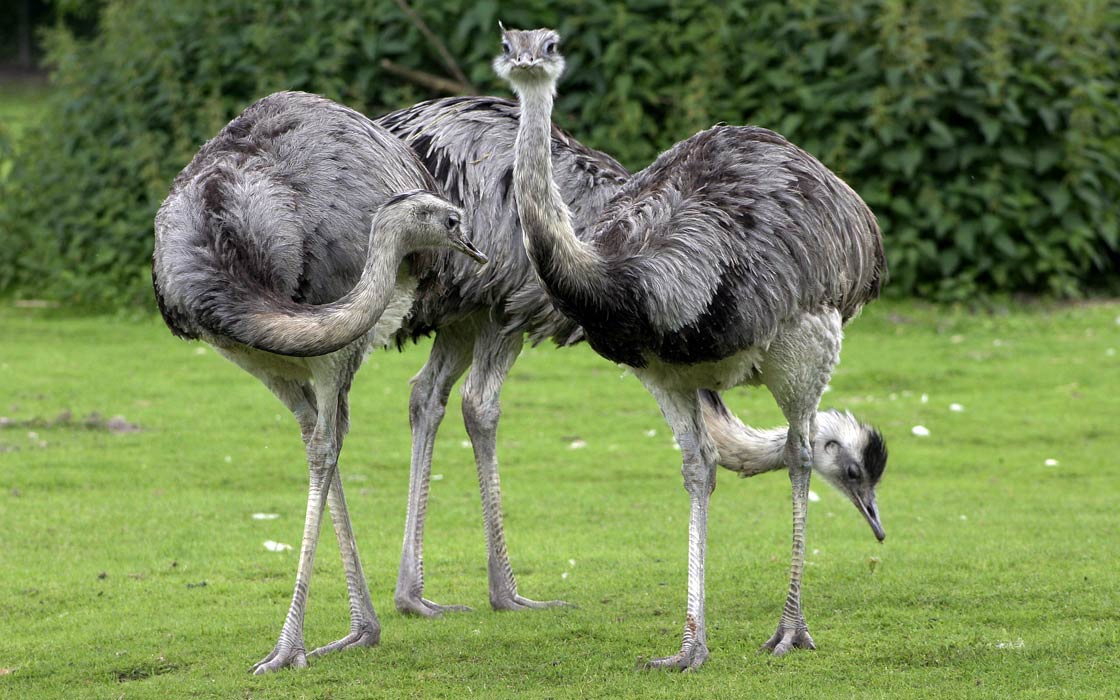The photograph features three ostriches with long, S-shaped necks, displaying different shades of gray feathers, standing on a large, somewhat worn grassy field that is dotted with small white flowers. In the background, green trees and a large shrubbery with brown twigs protruding can be seen. The ostrich on the left is standing with its legs crossed, its neck turned to the left, appearing as the right side from our perspective. The middle ostrich is bent over, with its beak close to the ground, seemingly about to peck at something on the grass. The ostrich on the right stands tall, gazing directly at the camera. The ostrich in the middle also has a distinct black spot on the top of its head. The image is a realistic outdoor capture, with clear details of the ostriches' postures and surroundings.